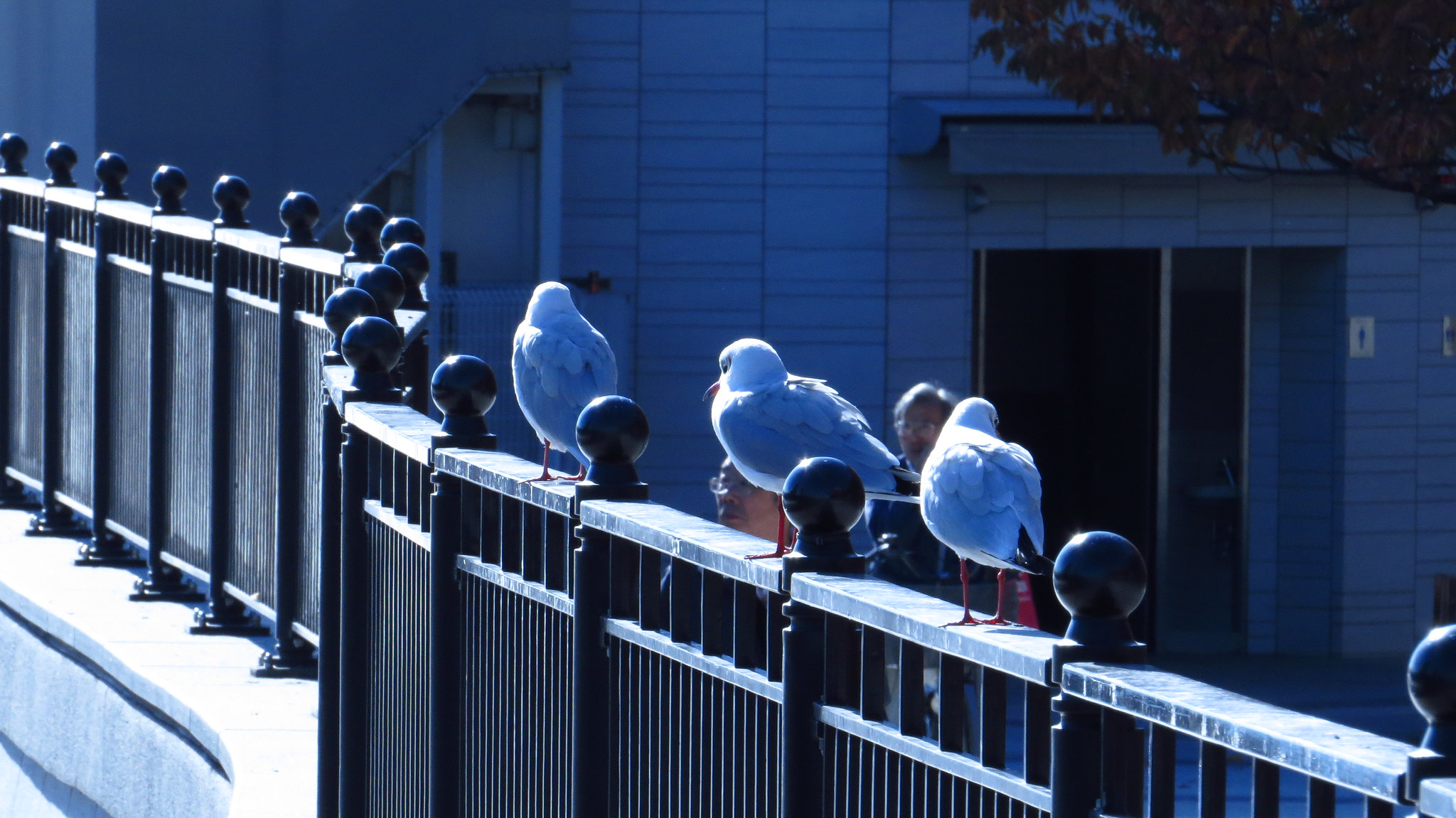In the photograph, a sunny day illuminates a scene featuring a black iron fence adorned with ball-shaped designs running across the top. This fence is erected on a small concrete wall, beyond which stands a white building with a layered brick or tile facade. Two older men, both with gray hair, glasses, and mustaches, are visible behind the fence. One man stands closer to the fence, while the other is positioned further back. Both appear to be intently observing the fence. Perched in a single line atop the fence are three fluffy seagulls. These birds have distinct orange legs and feet, white heads, and gray and white plumage with some slate-blue and black-tipped wing feathers. Their orange beaks also feature black tips. The scene is accented by tree branches and outdoor elements, suggesting the presence of a nearby body of water, which is potentially indicated by the safety barrier and overall setting. The detailed backdrop includes a glimpse of large building amenities like bathroom signs, indicating the area could be near public or office spaces.